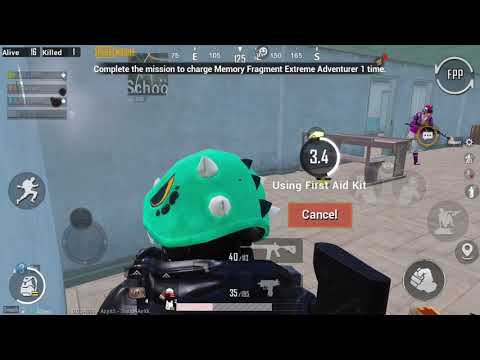This image is a screenshot from a combat-themed video game. It shows a scene set indoors, featuring light blue walls and shiny beige or cream-colored tile floors. In the forefront, a character from behind is seen wearing tactical gear and a distinctive green helmet. The helmet is adorned with an eye painted on it and has both black and white spikes protruding from it, resembling dinosaur spikes. Just the shoulder of this character in tactical, black bulletproof apparel is visible. 

The heads-up display (HUD) includes several game icons, like a fist, a running man, and a backpack in circles. At the top left corner, it displays "alive six killed one," while the top center reads, "Complete the mission to charge Memory Fragment Extreme Adventure one time." The foreground character is also shown with labels indicating the use of a "first aid kit," with an option to "cancel."

In the background, another character wearing purple gear and a matching purple helmet is visible, seemingly emerging from a doorway. This distant character appears to be holding an assault rifle, though one caption suggests it might be mistaken for a mop or broom due to the image being blurry. The game mode notation "FPP" (First-Person Perspective) is circled and located at the right side of the image.